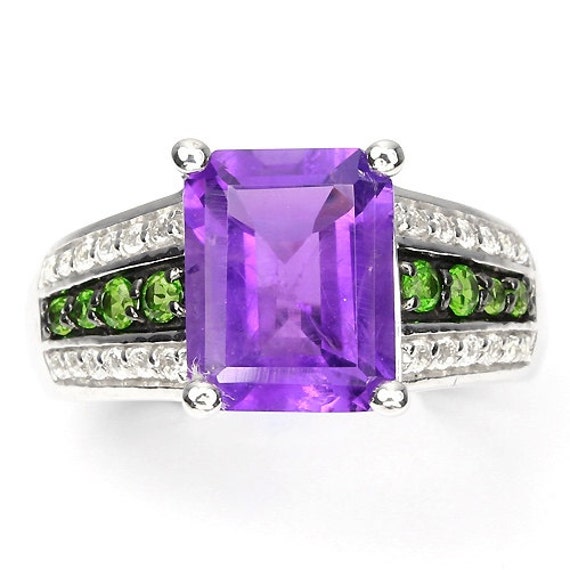The image showcases an extreme close-up of a ring, positioned on a white background likely for a retail or auction display. The ring features a prominent rectangular-shaped purple gemstone, possibly an amethyst, centrally placed and directly facing the viewer. This gemstone is set with small round clasps at each of its four corners. Surrounding the central purple stone, the ring is designed with three distinct rows. The middle row is adorned with green stones set against a dark black background, which encircle the circumference of the ring. Flanking this central row, the top and bottom rows are embedded with clear, diamond-like stones that also extend around the entire ring. The overall band of the ring appears to be of a white-gold color, emphasizing its luxurious design.